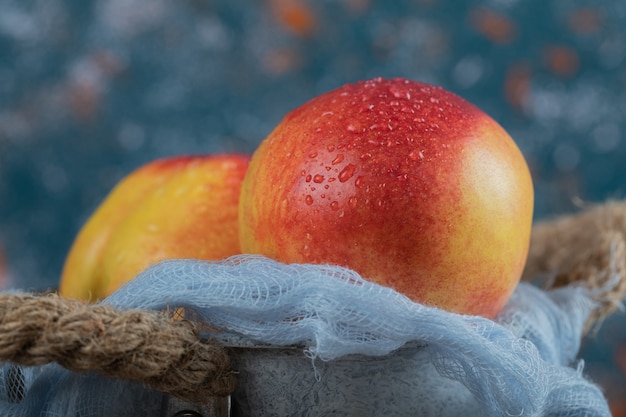The image showcases two freshly picked and washed peaches, glistening with water droplets on their vibrant, fuzzy skins. The ripe fruits, characterized by their spherical shape and rosy-red hues mingled with shades of yellow and orange, are nestled side-by-side in a basket or metal bucket. The container, which features braided and slightly frayed rope handles, is lined with a loose white gauze-like fabric, akin to medical gauze or cheesecloth. The background of the image is a soft blur of blue, white, and orange colors, providing a pleasing contrast to the richly colored peaches.